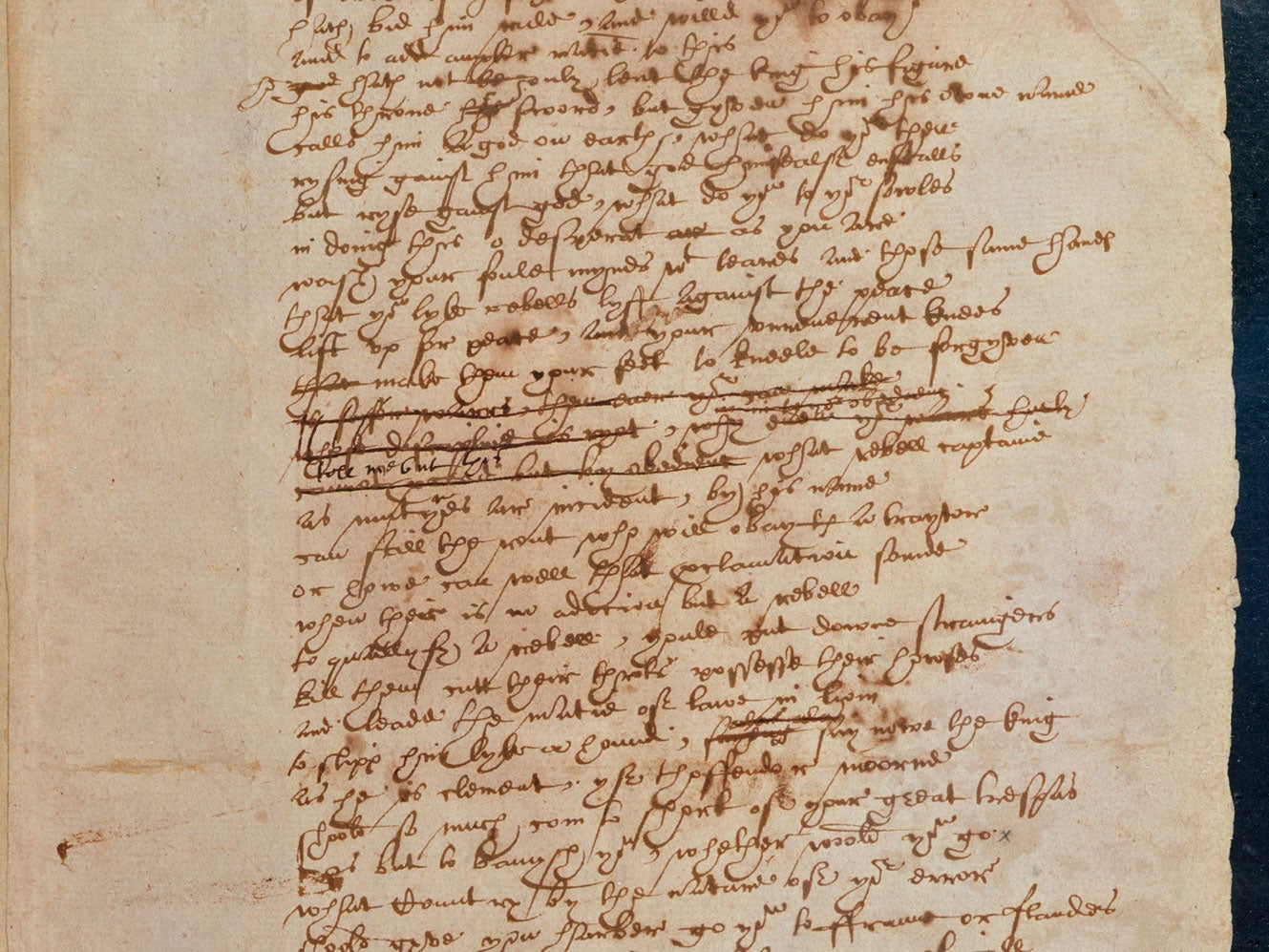The image features an aged sheet of parchment paper, displaying an extensive paragraph of dense, cursive writing in dark brown ink. The parchment, yellowed and creased with age, occupies the central third of the image, with noticeable blank margins on the left and a slightly narrower space on the right. The edges of the parchment are tattered and irregular, suggesting it may have been torn from a larger piece. The text, handwritten in a small, elegant script, is difficult to decipher and may be in a different language. Some lines are underlined, and there are crossed-out sections, indicating possible corrections. The parchment appears to rest on a black surface, likely a black table, which is visible as a thin vertical strip along the right edge of the image.